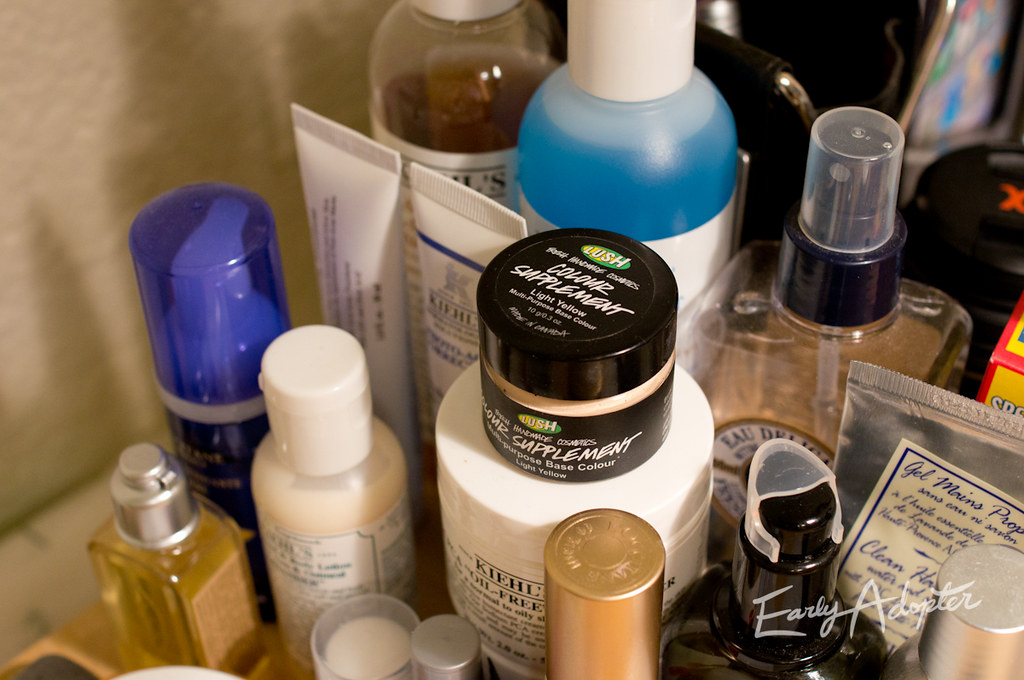This photograph showcases an assorted collection of bathroom products, meticulously arranged to highlight their diversity and utility. At the center of the composition, a prominent small jar with a black lid, labeled as a color supplement, captures immediate attention. Directly behind this central jar stands an opaque white container filled with a striking blue liquid. To its left, there is a brownish-yellow liquid displayed in another container.

In the foreground of these liquids, two tubes of creams are prominently situated, their labels partially visible. Just ahead, a blue-top container, likely a foaming cleanser, is accompanied by a bottle featuring a white cap, presumably a lotion. Further to the right, a small sprayer bottle, possibly containing cologne, is observed.

Returning focus to the central jar, it is placed atop a container branded with "Kiehl's Oil-Free" partially visible on its label. A subtle watermark reading "Early Adopter" is positioned at the bottom-right corner of the image, adding a modern touch. Below this, another container with a spray head can be glimpsed, enriching the composition with an additional layer of functionality.

The arrangement provides a vivid snapshot of a well-curated personal care collection, suggestive of a thorough grooming routine.